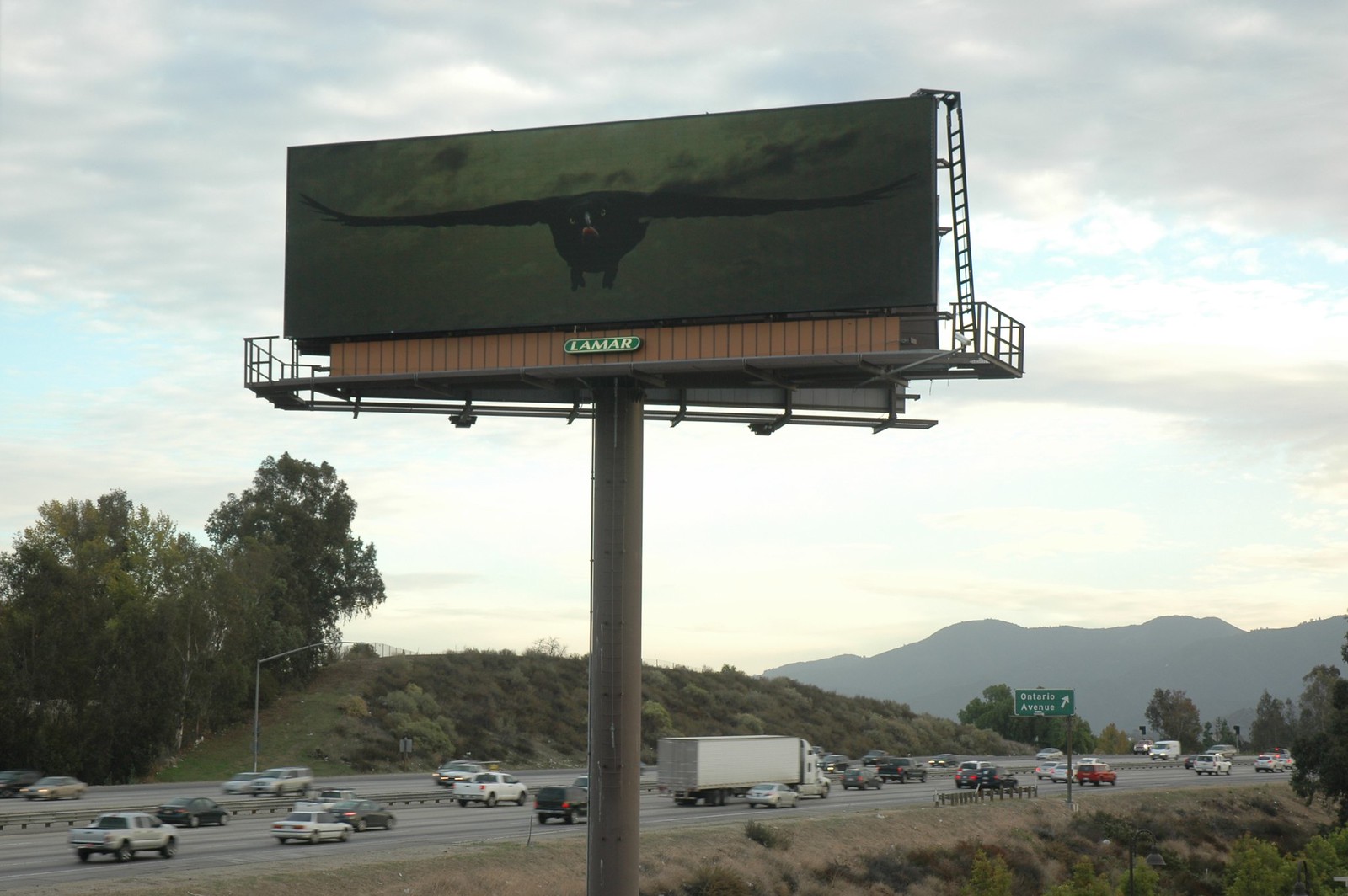This is a color photograph depicting a busy six-lane highway—three lanes in each direction—teeming with cars and trucks traveling both ways. In the foreground, a large cylindrical steel pole supports a big rectangular green billboard. The billboard features a bird flying toward the camera, wings outstretched and legs dangling, with the word "LAMAR" written in large white letters below the bird. To the right of the highway, there is a cluster of green trees and a small hill. More trees form a dense line above this area, and beyond that, another larger hill can be seen. In the background, the sky is mostly gray with some light cloud cover, and there are distant mountains adding depth to the scene.